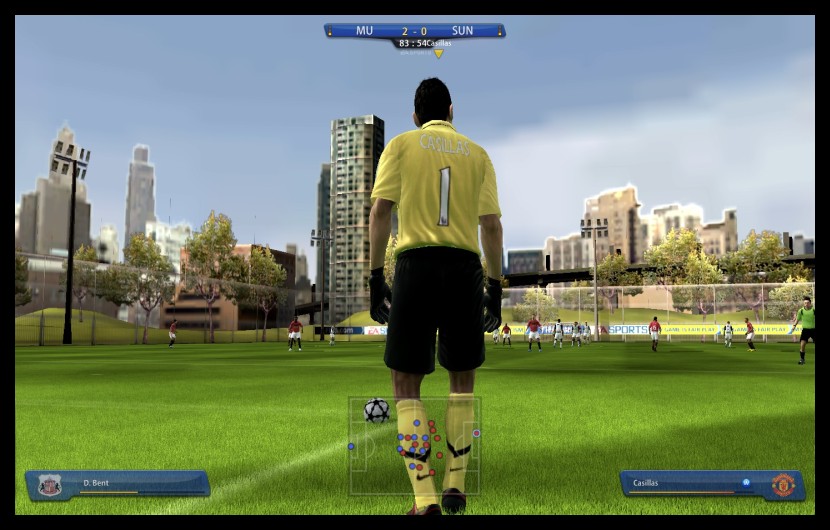In this still from a football (soccer) match, we observe a player from behind, standing on the field with a striking urban backdrop. The horizon showcases a cityscape dotted with towering buildings, while stadium floodlights on the left hint at preparations for a potential night game. Above, the sky is blanketed with dark, brooding clouds that create a dramatic atmosphere. 

From the midpoint right along the horizon, advertising boards typical of a professional pitch are visible, suggesting a high-stakes environment. The player, a person of color, wears a vibrant yellow jersey emblazoned with the number "1" in white, black shorts, and knee-length yellow socks accented with stripes. 

In the bottom corners of the image, blue information blocks display team logos and player details, adding a touch of modern sports broadcasting to the scene. This detailed backdrop and the player's poised stance hint at a moment of anticipation and readiness in the game.